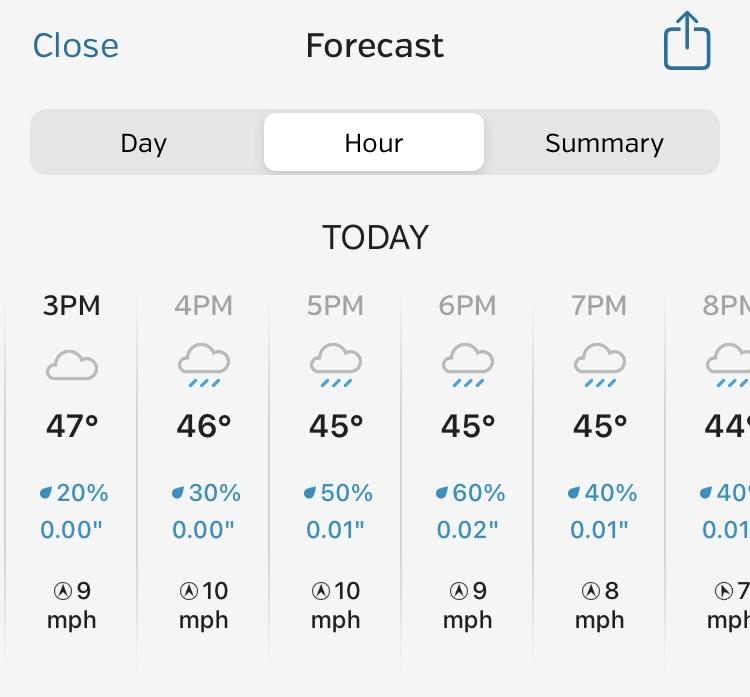In the image, we see a detailed weather forecast page. The top of the page displays navigational options: "Close," "Forecast," "Share," "Day," "Hour," and "Summary." The "Hour" option is currently selected. 

The forecast provides hour-by-hour details for today starting at 3 p.m. At 3 p.m., the temperature is 47°F with a humidity level of 20% and a wind speed of 9 miles per hour. 

At 4 p.m., the temperature drops slightly to 46°F, humidity increases to 30%, and the wind speed rises to 10 miles per hour. 

By 5 p.m., the temperature further decreases to 45°F, while the humidity climbs to 50% and the wind speed remains steady at 10 miles per hour.

At 6 p.m., the temperature holds at 45°F, but humidity grows significantly to 60%, and the wind speed reduces to 9 miles per hour.

At 7 p.m., the temperature is consistent at 45°F, with humidity decreasing to 40% and the wind speed continuing to drop to 8 miles per hour.

Finally, by 8 p.m., the temperature slightly lowers to 44°F, with the humidity holding at 40% and the wind speed reducing further to 7 miles per hour. 

This meticulous breakdown of weather conditions helps in planning activities throughout the evening.